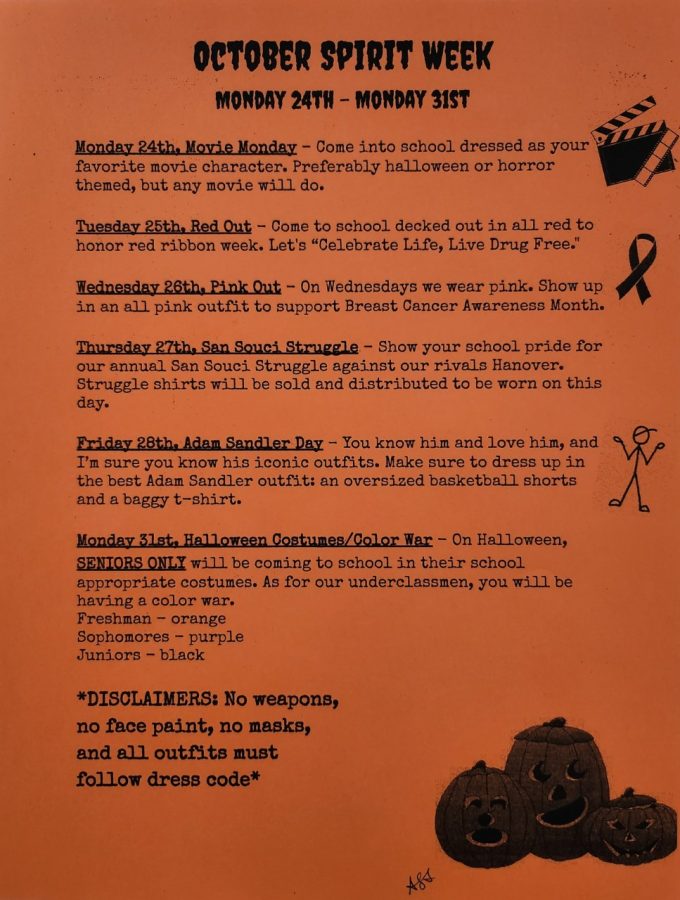This detailed and vibrant flyer, set against a solid burnt orange background, announces October Spirit Week, running from Monday the 24th to Monday the 31st. The event title, "October Spirit Week," is prominently displayed in black oozing text at the top center. Beneath this header, the schedule and themes for each day are laid out, accompanied by relevant illustrations along the right side.

- **Monday, the 24th: Movie Monday:** Students are encouraged to come to school dressed as their favorite movie characters, with a preference for Halloween or horror themes, although any movie character is acceptable.
  - *Illustration:* A movie clapperboard.

- **Tuesday, the 25th: Red Out:** In honor of Red Ribbon Week, everyone is encouraged to wear red to celebrate a life lived drug-free.
  - *Illustration:* Three pumpkins with different facial expressions— the middle pumpkin has crescent-shaped eyes and a turned mouth, the smaller pumpkin has diamond eyes, a jagged mouth, and a triangle nose, and the left pumpkin has sad eyes with a circular mouth and an angry face.

- **Wednesday, the 26th: Pink Out:** Students are asked to show up in all pink outfits to support Breast Cancer Awareness Month.
  - *Illustration:* A small breast cancer ribbon.

- **Thursday, the 27th: San Socio Struggle:** Show school pride for the annual San Socio Struggle against rivals Hoover Hanover by wearing special struggle shirts, which will be sold and distributed beforehand.
  - *Illustration:* Three pumpkins with different faces and different eyes.

- **Friday, the 28th: Adam Sandler Day:** Students should dress up in iconic Adam Sandler outfits, typically consisting of oversized basketball shorts, a baggy t-shirt, and a baseball cap.
  - *Illustration:* A stick figure in an Adam Sandler-inspired outfit.

- **Monday, the 31st: Halloween Costumes/Color War:** Seniors are permitted to wear school-appropriate Halloween costumes. Underclassmen are to participate in a Color War by wearing distinct colors—freshmen wear orange, sophomores purple, and juniors black.
  - *Illustration:* A stick figure with a baseball cap for Adam Sandler Day, a ribbon next to Cancer Awareness, and a movie clapperboard for Movie Monday.

The flyer also includes bold text disclaimers at the bottom: "No weapons, no face paint, no masks, and all outfits must follow the dress code."